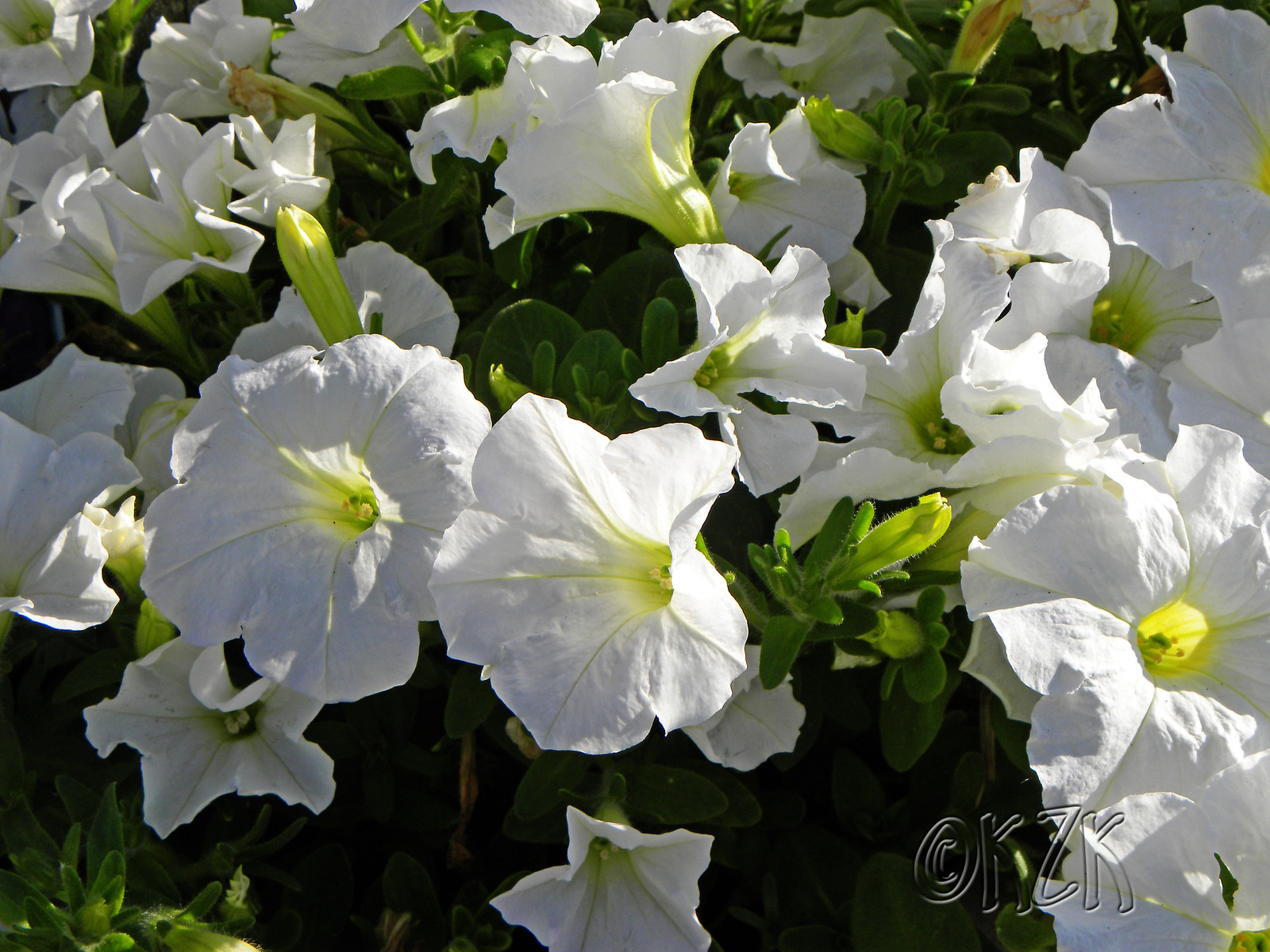The photograph captures a dense cluster of large white flowers, each resembling tissue paper with deeply recessed yellowish-green centers sprinkled with tiny orange specks. These flowers grow on a bush, filling the entire frame and interspersed with green leaves. The sunlight, casting brighter light on the right side, illuminates the delicate petals and creates darker, shadowed areas underneath the foliage. The background appears dark, enhancing the brightness of the white blooms. In the bottom right corner, there is a distinctive watermark with the copyright symbol and the letters "KZK" in a hand-drawn, transparent outline.